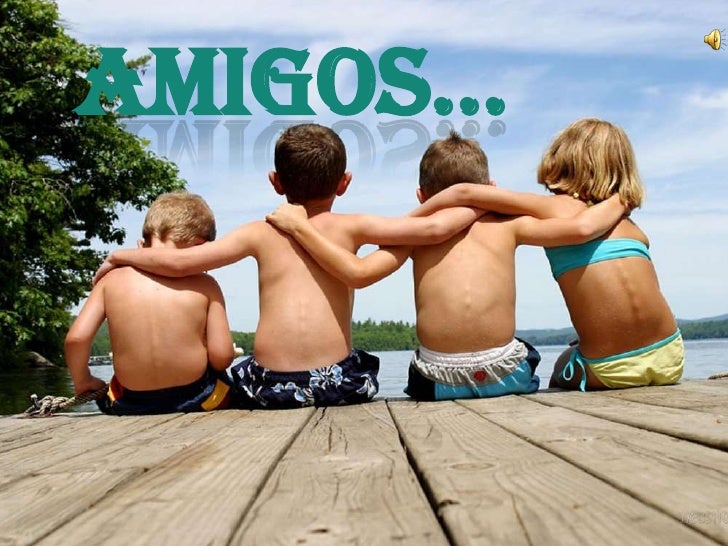The photograph, titled "Amigos..." in dark bold green letters with a reflection effect, captures a serene moment on a dock by the lake. Four children, three boys on the left and one girl on the right, all white, are sitting side by side with their backs to the camera. They are interlocking arms, each child’s hand resting on the shoulder of the next, symbolizing a strong bond of friendship. The boys sport various swim trunks, including flower-patterned ones on the middle-left boy, while the girl on the right wears a two-piece blue and yellow bathing suit. The background features a picturesque view of the water with a blue sky, light clouds, and a distant tree line, adding a tranquil ambiance to the scene. A wooden dock beneath them and some foliage on the left edge complete the frame. Additionally, a small gold speaker symbol appears at the upper right corner of the image, adding an unexpected modern touch.